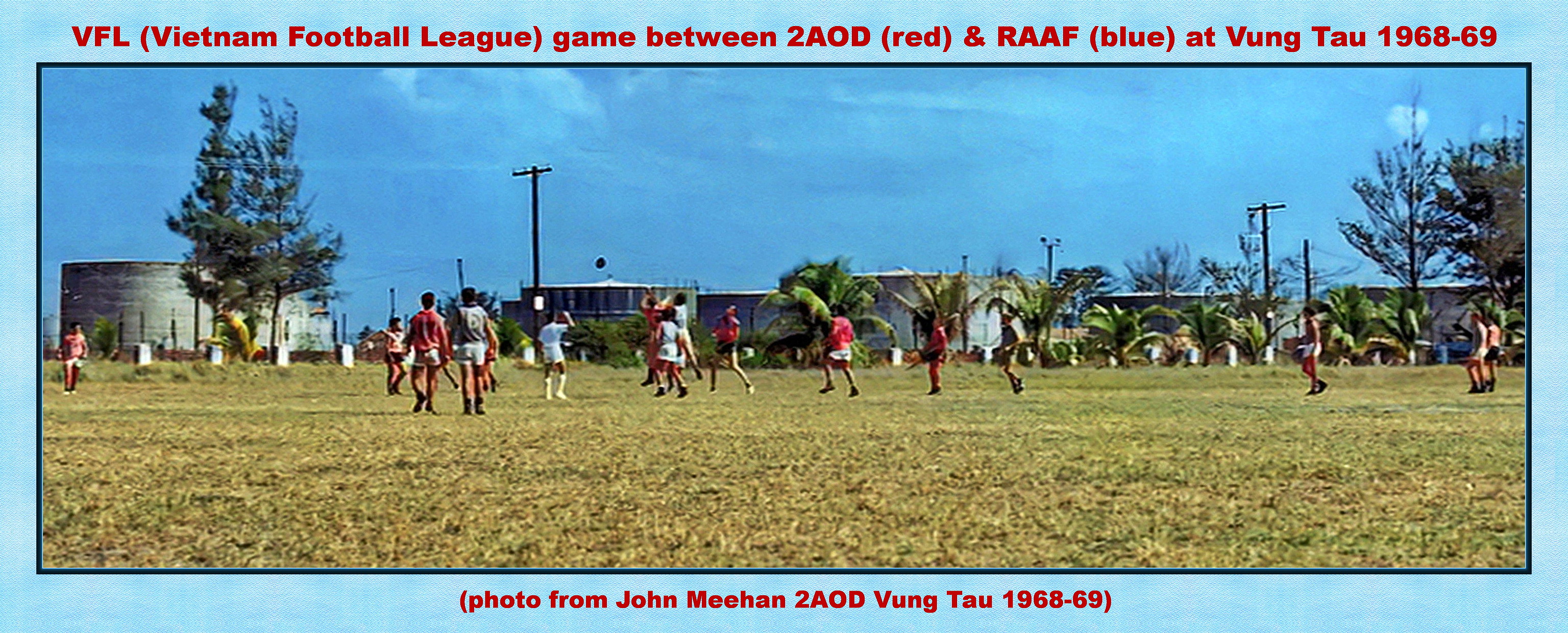This poster, spanning a very wide rectangular frame, captures an outdoor scene from an intriguing historical backdrop: a football (soccer) game of the Vietnam Football League. The light blue sky forms the serene background for this nostalgic image. Detailed in vivid red font at the top, the text reads: "VFL (Vietnam Football League) game between 2AOD (red) and RAAF (blue) at Vung Tau, 1968-69." Below this, in a smaller yet matching red font, there's a credit: "Photo from John Meehan, 2AOD, Vung Tau, 1968-69."

The bottom half of the image reveals a slightly browned grass field where teams in orange and white gear are actively playing soccer. The scene is peppered with rural elements: distant buildings, telephone poles, and scattered trees juxtaposed against the light blue sky, indicating a daytime setting. Players, possibly air force members judging by the context, are either standing or running across the field, immersing us in the vibrant atmosphere of this historical match. The visual palette includes hues of light blue, red, green, tan, yellow, and orange, harmonizing with the image’s nostalgic and dynamic essence.